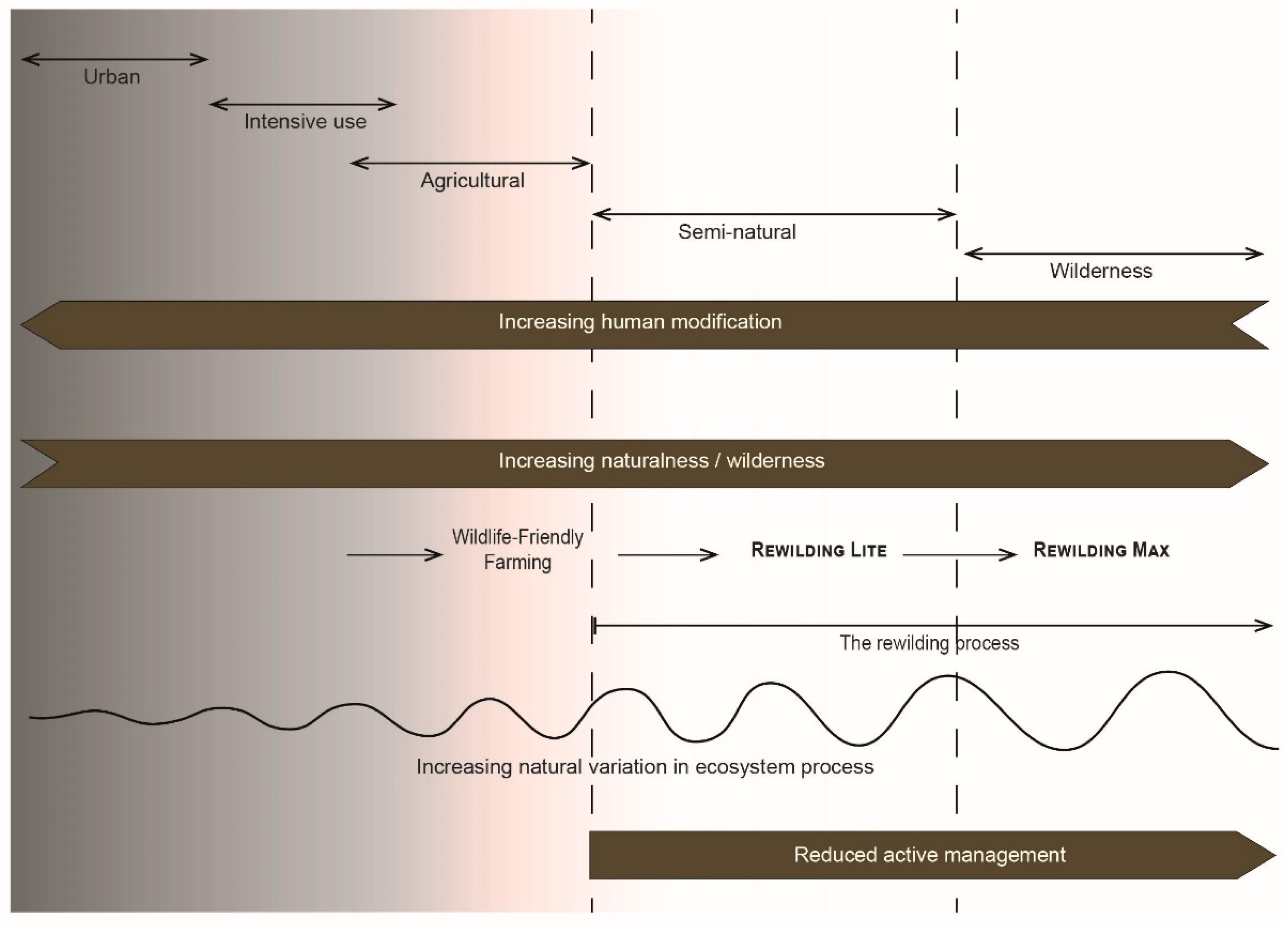The diagram features a gradient background transitioning from grayish-purple on the left to white on the right, representing a spectrum. From the top left to the middle right, there are multiple horizontal arrows, each labeled sequentially: "Urban," "Intensive Use," "Agriculture," "Semi-Natural," and "Wilderness." These arrows are aligned beneath a brown banner labeled "Increasing Human Modification" pointing to the left, and a corresponding banner labeled "Increasing Naturalness/Wilderness" pointing to the right.

Beneath these elements is a secondary section showcasing three right-pointing arrows labeled "Wildlife-Friendly Farming," "Rewilding Lite," and "Rewilding Max," followed by a significant arrow labeled "Rewilding Process." Underneath this section lies a wavy line stretching across the image labeled "Increasing Natural Variation in Ecosystem Process," with the text "Reduced Active Management" beneath it.